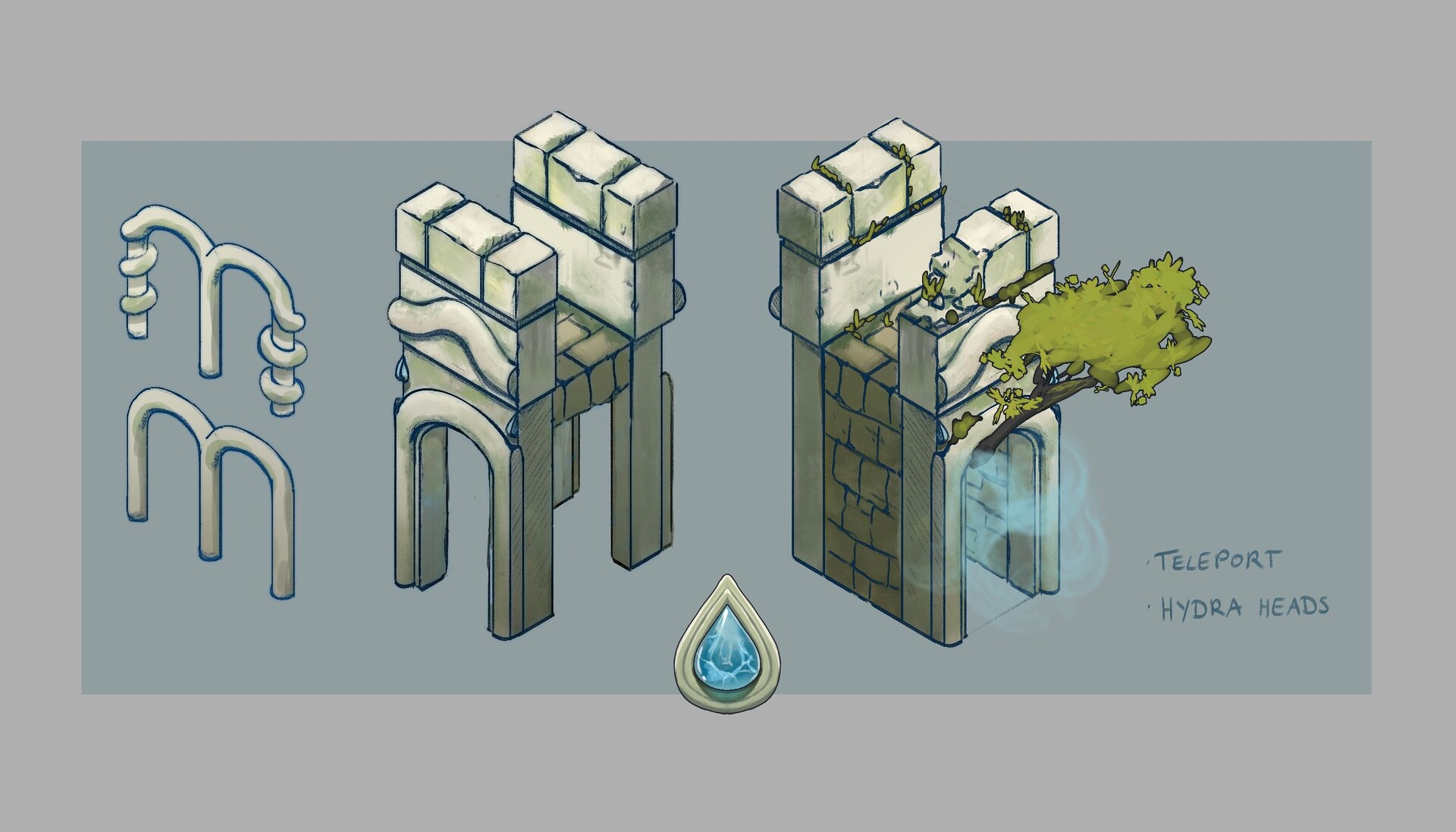The image consists of three sequential drawings that collectively illustrate the construction and completion of a teleport-like bridge structure. The rectangular image, approximately five inches wide and three inches high, is surrounded by a dark gray border, with the top and bottom edges being thicker than the sides. Within this border, there is a slightly green, grayish-blue inner rectangle. 

The first drawing on the far left features two M-shaped stone arches with spiral corkscrew designs on both sides. Moving right, the second drawing depicts a more developed structure resembling a bridge made of square tan and brown bricks, with a curved bottom. 

The third drawing on the right shows the completed bridge with the arches fully assembled, aged, and integrated with nature—a tree limb grows out from beneath the structure, and blue smoke emanates from it. The once-solid bricks are now crumbling with vegetation creeping through. At the very bottom center of the image, a teardrop-shaped blue gem with a light greenish-gray encasement extends slightly into the border. 

In the bottom right corner, there's a handwritten note that says "Teleport Hydra Heads." The consistent style and overlapping illustrations create a cohesive, detailed depiction of this mystical teleportation bridge.